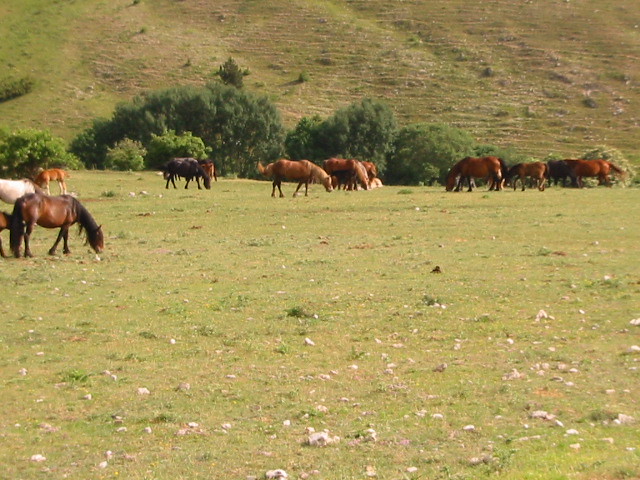The outdoor color photograph captures a serene prairie scene bathed in bright overhead sunlight, which eliminates any hard shadows. The expansive grass field spanning the foreground is dotted with white stones and possibly some scattered leaves or bones. The grass is short and varies in shades of green, interspersed with gray patches.

In the background, a group of approximately 10 to 12 horses is seen grazing. These horses display a range of colors, mostly shades of brown with some dark manes and legs, one black, and another white one positioned farther to the left. They are scattered across the field, with clusters of five here, three there, and smaller groups or solitary horses further out.

A line of variously sized green trees, about a story tall, sits behind the grazing horses. Beyond the tree line, a gently sloping hill stretches up to the edge of the frame. The hill features a mix of green and brown grass, scruffy patches, and a few exposed striated rocks, giving it a rugged texture that complements the tranquil atmosphere of the prairie. There are no printed words or texts in the image, drawing the focus entirely on the natural beauty of the scene and the harmony of the grazing horses in the landscape.